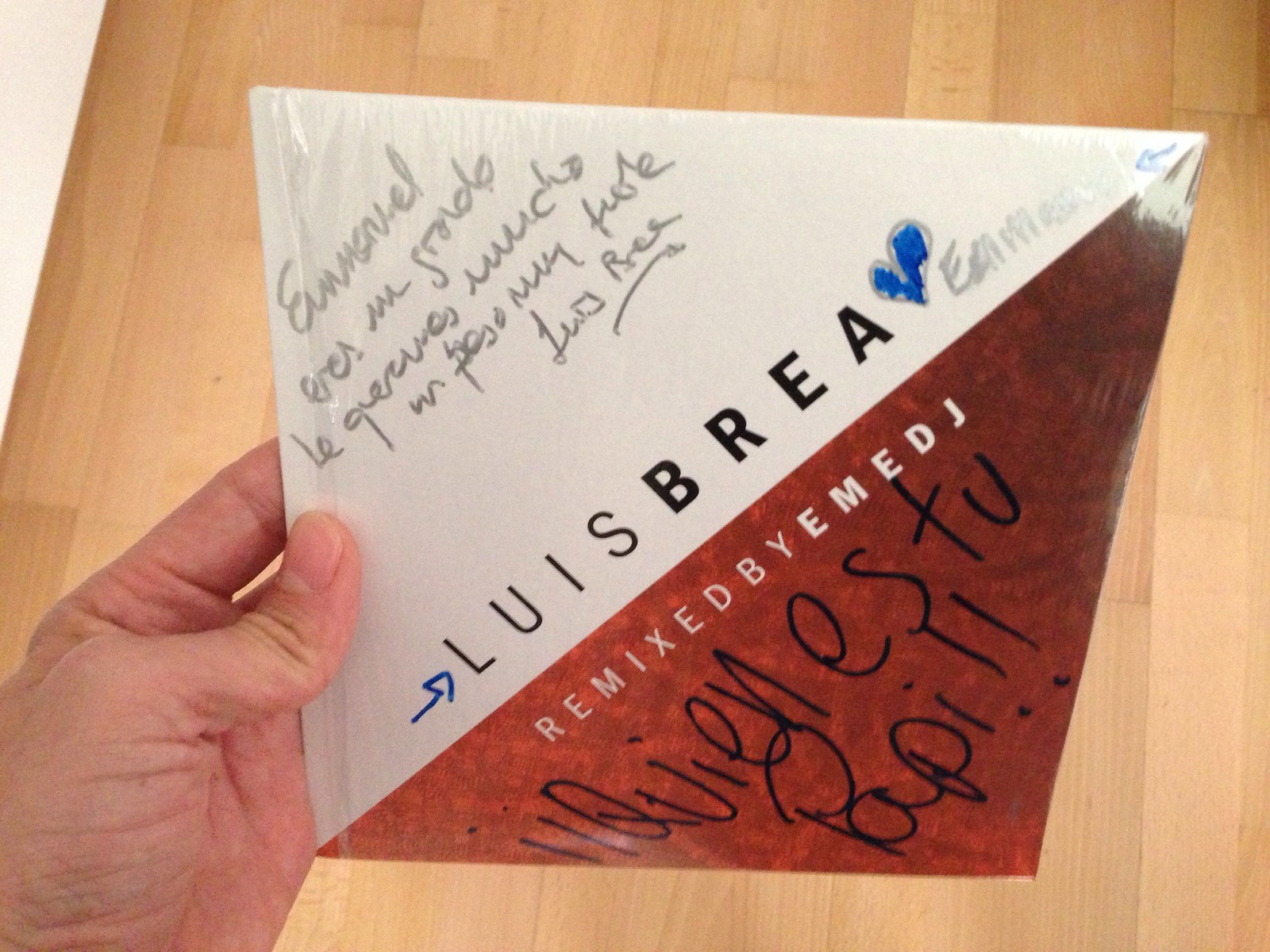The image showcases a slim, square CD or vinyl cover that appears to be autographed. The cover is diagonally divided; the top left section is white, featuring the printed name "Luis Brea," while the bottom right section has a red and black mixed background, adorned with additional handwriting. In the upper left corner, there is some handwritten text in silver marker that seems to be in Spanish, beginning with "Emanuel Edis," though the rest is not fully legible. Directly under "Luis Brea," it states "Remixed by EMEDJ," with further black marker inscriptions below. The artwork also includes blue arrows drawn on either side of "Luis Brea" and a blue-colored heart with the name "Emanuel" next to it. Another handwritten note in black marker reads "kien es tu papi." The cover is being held up by a Caucasian hand against a backdrop of a brown wooden floor.